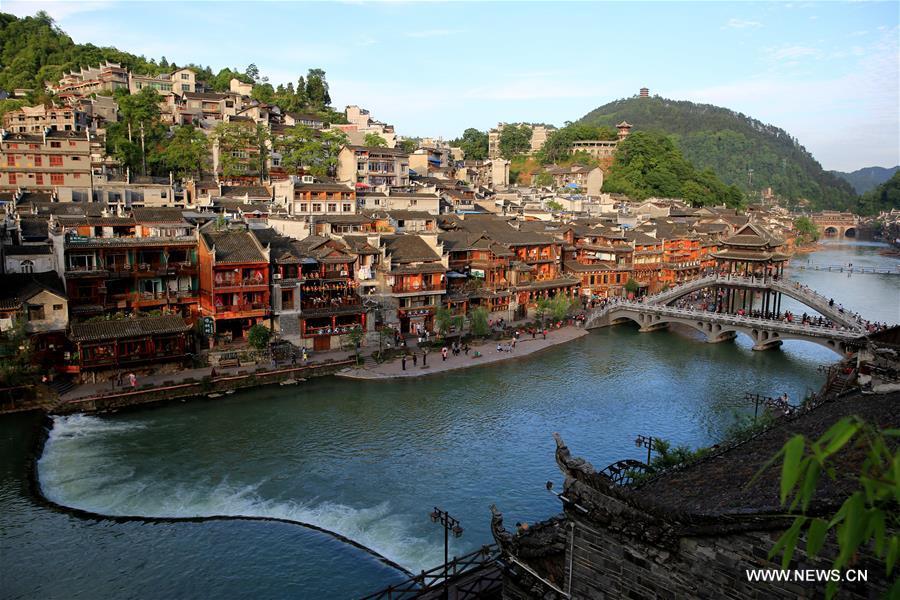This outdoor daytime photograph, featuring a white watermark reading "www.news.cn" at the bottom right, captures a picturesque cityscape on a river's edge. The scene focuses on a densely populated town with rows of multi-storied houses and buildings in shades of brown, white, tan, and orange, closely packed together along the steep, grassy hillside. The river, a beautiful light green to blue hue, runs from the lower left corner to the right edge of the image, intersected by a bridge that connects the town to the opposite bank. This far bank features a terrain of ground, dirt, and scattered plants. People can be seen walking along the riverbank in the foreground. The landscape extends upwards to a lush, green mountain area, adding a backdrop of natural beauty. The overall atmosphere, reminiscent of Italian or possibly Chinese architecture, vividly portrays a harmony between the man-made structures and the natural surroundings under a clear sky.